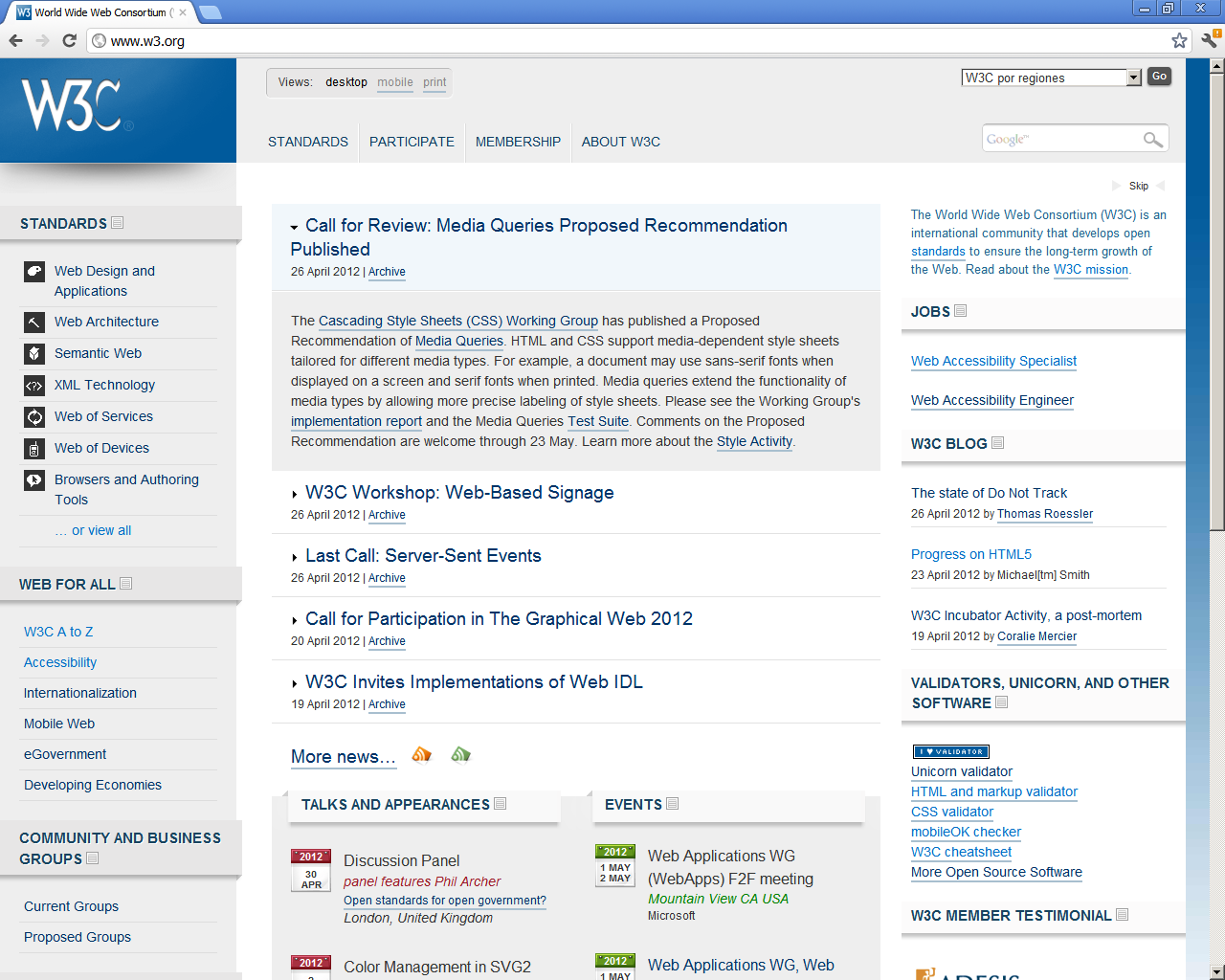The image depicts a webpage from the World Wide Web Consortium (W3C) website. The interface features a predominantly gray background with black lettering. At the top, there is a small blue square logo with "W" and "S" in white. A search bar at the top contains the URL "www.w3.org," leading to a page displaying several sections and links.

On the left side, a prominent blue banner displays the W3C logo, followed by a gray area with blue subheadings. These subheadings include "Standards," "Web Design and Applications," "Web Architecture," "Semantic Web," "XML Technology," "Web of Services," "Web of Devices," "Browsers," and "Authoring Tools." An icon in black and white is adjacent to a blue link labeled "View All."

Additional sections below include "Web for All" in dark blue, with related topics such as "Accessibility," "Internationalization," "Mobile Web," "E-Government," and "Developing Economies" detailed in lighter blue.

A darker gray banner follows, labeled "Community and Business Groups" in dark blue, with links to "Current Groups" and "Proposed Groups" underneath. In the center, a section labeled "Views" provides options for desktop, mobile, or print views, with "Desktop" highlighted in black. Below this, links to "Standards," "Participate," "Membership," and "About W3C" are displayed in blue.

On the right side, another search bar shows a query for "W3C for regionals." Below, a list features a call for review of "Media Queries Proposed Recommendation" dated April 26, 2012, and a clickable blue "Archive" link.

A paragraph in black text contains clickable blue links, highlighting recent W3C activities and events such as "W3C Workshop," "Web-based Signage," "Last Call Server Sent Events," and "Call for Participation in the Graphical Web 2012." Dates and additional "Archive" links are included.

At the bottom, a "More News" link in blue is followed by "Top Appearances," featuring calendar icons in red and white with dates in black. Events listed include discussion panels on "Color Management" and "Web Applications WG Web."

Lastly, a right-side menu lists various clickable topics in blue, offering further navigation through the website’s content.